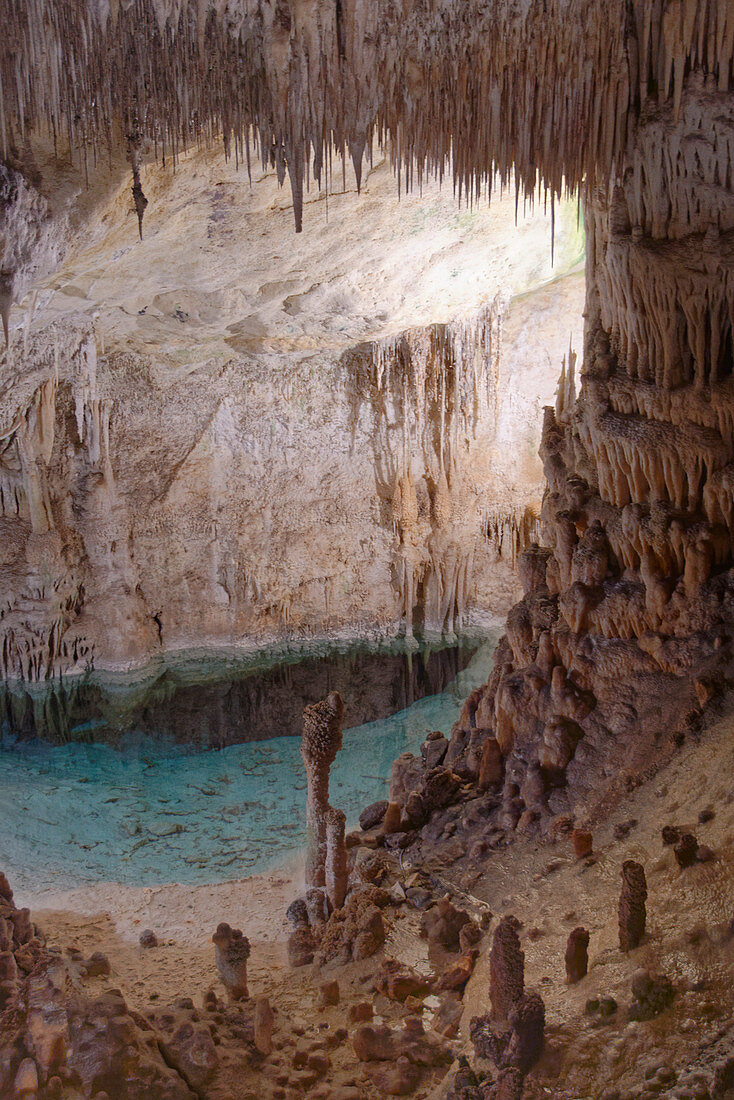The photograph showcases the intricate interior of a massive cavern, possibly a salt mine, illuminated by a shaft of bright sunlight streaming through a large opening on the right. The cavern's ceiling is adorned with hundreds, if not thousands, of sharp, needle-like stalactites and stalagmites, bearing a reddish-brown hue. The walls are lined with rocky formations and patches of cream-colored dirt, with parts appearing to have a melted, smooth texture. Toward the back, the cavern wall shifts to smoother surfaces with creams and browns. The floor is a striking mix: near the front lie clusters of fallen rocks and dirt, while a section further in reveals a mysterious blue area, possibly water, turning black with depth, adding an enigmatic touch to the cavern's grandeur.